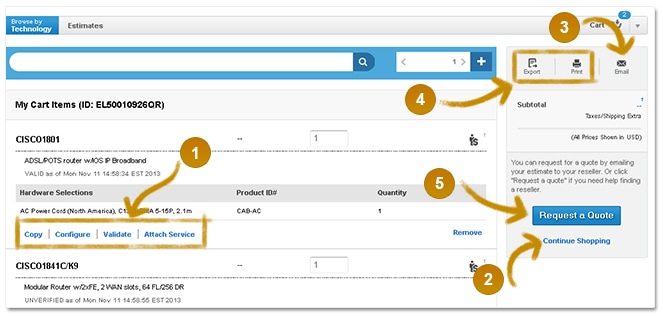The image appears to be an annotated and somewhat aged, grainy screenshot from a how-to guide. The background color is primarily white. At the top of the screen, there is a navigation bar. From left to right, the bar consists of a blue box labeled "Browse by Technology" followed by a long gray box titled "Estimates." The gray box stretches across to the right and displays a partially obscured blue oval with the number "2," indicating two items in the cart.

Several annotations, rendered in a gold-brown color, are present throughout the image. One annotation, labeled "3" in a circle with an arrow, points to an email icon positioned below another card-like section. Directly below this card, there's a blue box containing a search bar. Beneath the search bar, the text reads: "My Cart Items ID: EL50010926 QR, Cisco 1801." Following this, there is a box with the quantity "1" and an adjacent, unreadable icon. Accompanying text describes a "DSL POTS Router with IOS IP Broadband," valid as of "Monday, November 11, 14:58:34 EST 2013."

Further down, a gray box labeled "Hardware Selections" lists details like "Product ID" and "Quantity." The next item, "AZ Power Cord North America," is partially obscured by another arrow. The readable part of the product ID number cannot be discerned, and the quantity is "1." A boxed section below this area features blue text labeled "Copy, Configure, Validate, and Attach Service," accompanied by an annotation pointing to it and labeled "1."

Underneath this section, another product "Cisco 1841 C/K9" is partially visible but seems not to be the main focus. Another annotation labeled "2" in a circle points to "Continue Shopping" displayed in blue text at the bottom right.

On the right sidebar, from top to bottom, there's text reading "Export, Print, and Email," with an email icon annotated as "3." Below this, a form annotation points towards the "Export" and "Print" boxes. Further down, a subtotal is shown with a note about additional taxes and shipping costs, all prices listed in USD. There’s an option to "Request a Quote" facilitating contact with resellers, with annotated item "5" pointing to a blue box with white text that says "Request a Quote."